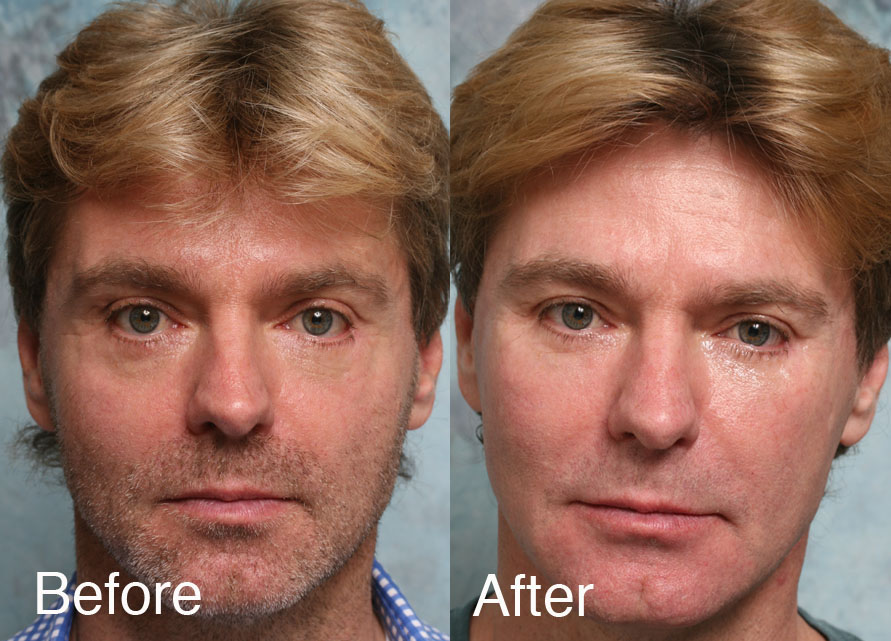This image is a side-by-side comparison of a young Caucasian man labeled "before" and "after." In the "before" picture on the left, the man has long, blonde hair, greenish-bluish eyes, and a scruffy beard. He is dressed in a white and blue collared shirt and is staring directly at the camera. Conversely, the "after" picture on the right shows the same man but with a considerably different look: he has shaved off his beard completely, his hair appears to be dyed a reddish color, and he has plucked eyebrows. He now wears a green t-shirt and looks slightly happier and less tired. The labels "before" and "after" are prominently displayed in white text on each respective photo.